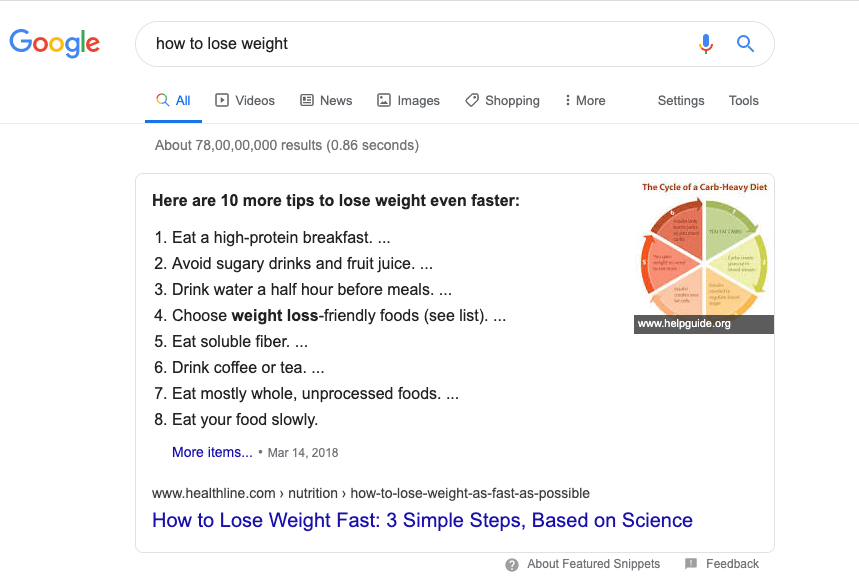This detailed caption captures the elements of a screenshot from a Google search page discussing weight loss methods:

The image depicts a screenshot of a Google search page. On the left side of the screen, the iconic Google logo is prominently displayed. Adjacent to it is the search bar, which contains the query "how to lose weight." To the right of the search bar, there are icons for a microphone and a search option. Below the search bar, a menu offers various options: the one currently selected and underlined is "All," followed by "Videos," "News," "Images," "Shopping," "More," and lastly "Settings and Tools."

Directly beneath this menu, the search results indicate approximately 780,000,000 results found in 0.86 seconds. The first result, highlighted in bold, is an article titled "Here Are 10 More Tips to Lose Weight Even Faster," accompanied by a brief list visible up to the eighth tip. The tips shown are: 
1. Eat a high-protein breakfast.
2. Avoid sugary drinks and fruit juice.
3. Drink water a half hour before meals.
4. Choose weight-loss-friendly foods.
5. Eat soluble fiber.
6. Drink coffee or tea.
7. Eat mostly whole, unprocessed foods.
8. Eat your food slowly.

Additionally, a sidebar on the right features a circular graph illustrating a carb-heavy diet. At the bottom of the image, there is a link titled "How to Lose Weight Fast: 3 Simple Steps Based on Science." This detailed visual captures the primary components of the search page, offering a comprehensive view of the content displayed.